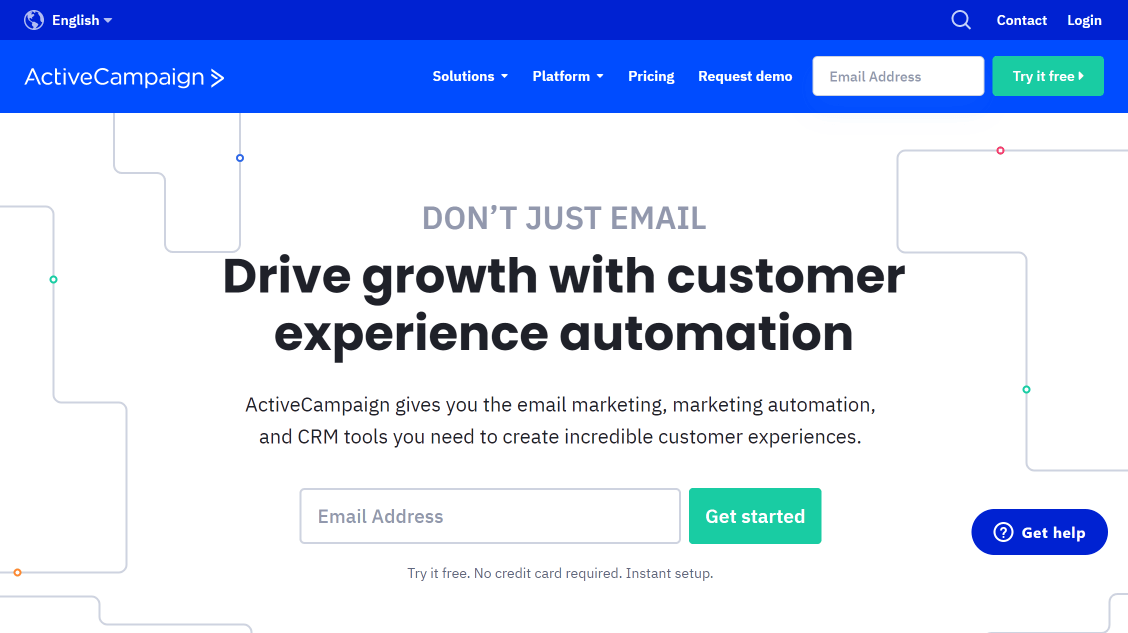The screenshot captures a web page with a structured layout. 

**Header:**
- A dark blue banner spans the top, featuring a globe icon and the word "English" on the left. 
- On the right, there's a magnifying glass icon beside the words "Contact" and "Login."

**Navigation Bar:**
- Beneath the header, a lighter blue strip stretches across the screen, marked by borders. 
- It contains navigation links: "ActiveCampaign" with a right-pointing arrow, "Solutions," "Platform," "Pricing," and "Request Demo."

**Main Section:**
- There's a primary call-to-action text box asking for an email address, paired with a prominent green button labeled "Try It Free."

**Body:**
- The main content area has a white background. 
- In the center, it reads "Don’t just email" in a moderate font, followed by a larger, bold tagline: "Drive growth with customer experience automation."
- Below this, in smaller text, the page explains: "ActiveCampaign gives you the email marketing, marketing automation, and CRM tools you need to create incredible customer experiences."

**Call-to-Action:**
- Another text box below invites users to enter their email address, accompanied by a green "Get Started" button in white text. 
- Additional smaller text reads: "Try it free, no credit card required, instant setup."

**Help Button:**
- To the right, a bluish-purple button displays a question mark icon and the words "Get Help" in white text.

**Design Elements:**
- The page is accentuated with lines and small circular motifs, adding dynamic visual interest.